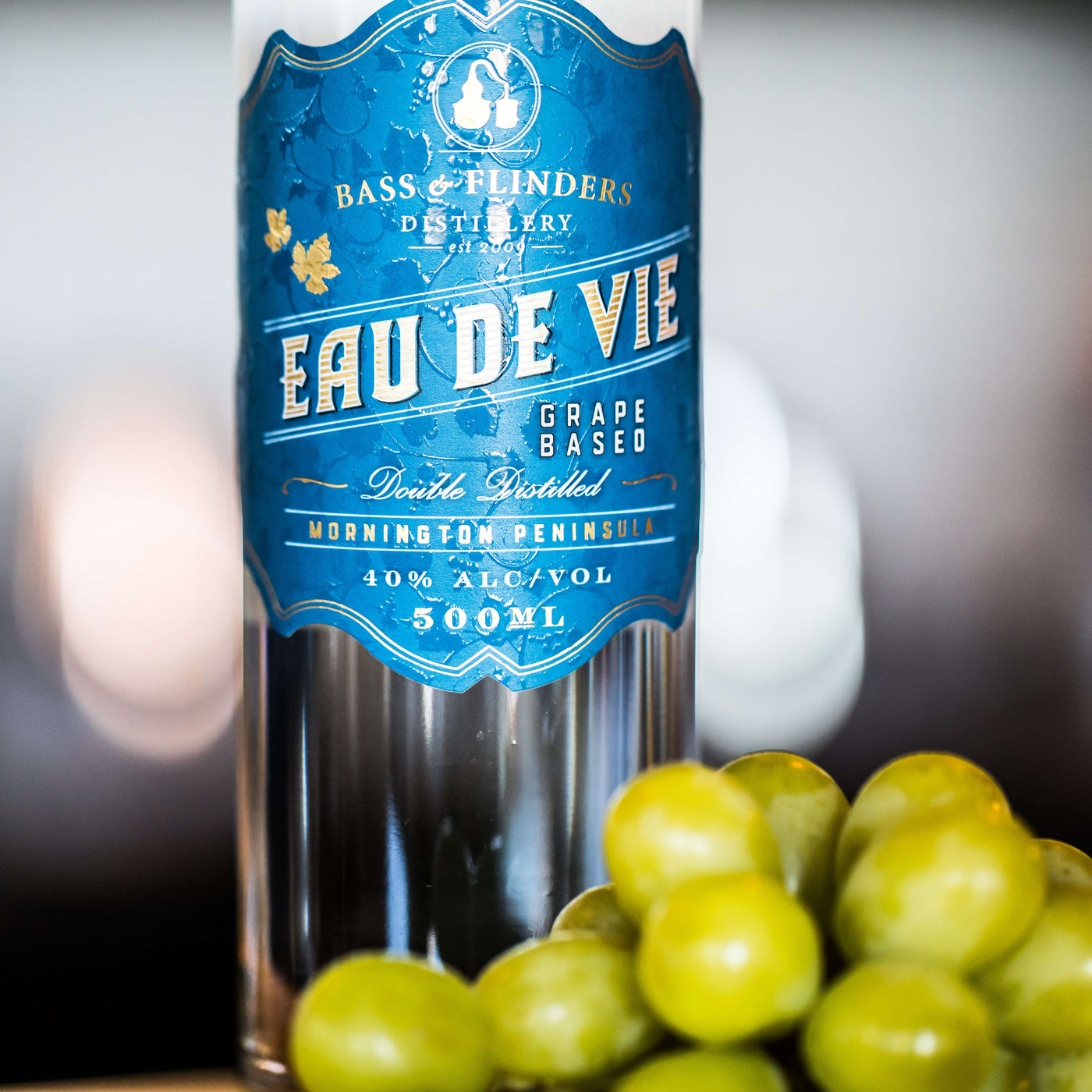The image showcases a close-up of a clear bottle of Eau de Vie, a grape-based, double-distilled alcohol from Bass and Flinders Distillery. The label, which is blue with dark embellishments of vines and leaves and a distinguishable white border, reads "Bass and Flinders Distillery, established 2009". The wine label also features two prominent gold-colored maple leaves near the top left. Further down, the label specifies the contents as "Eau de Vie," indicating its grape-based composition, "Mornington Peninsula," and "40% alcohol by volume, 500 milliliters." The background is blurred, transitioning from light gray at the top to nearly black at the bottom, with a peach-colored smear on the left side and a white smear on the right, possibly caused by lighting effects. In the foreground, there is a bunch of green olives or grapes adding a fresh element to the composition.